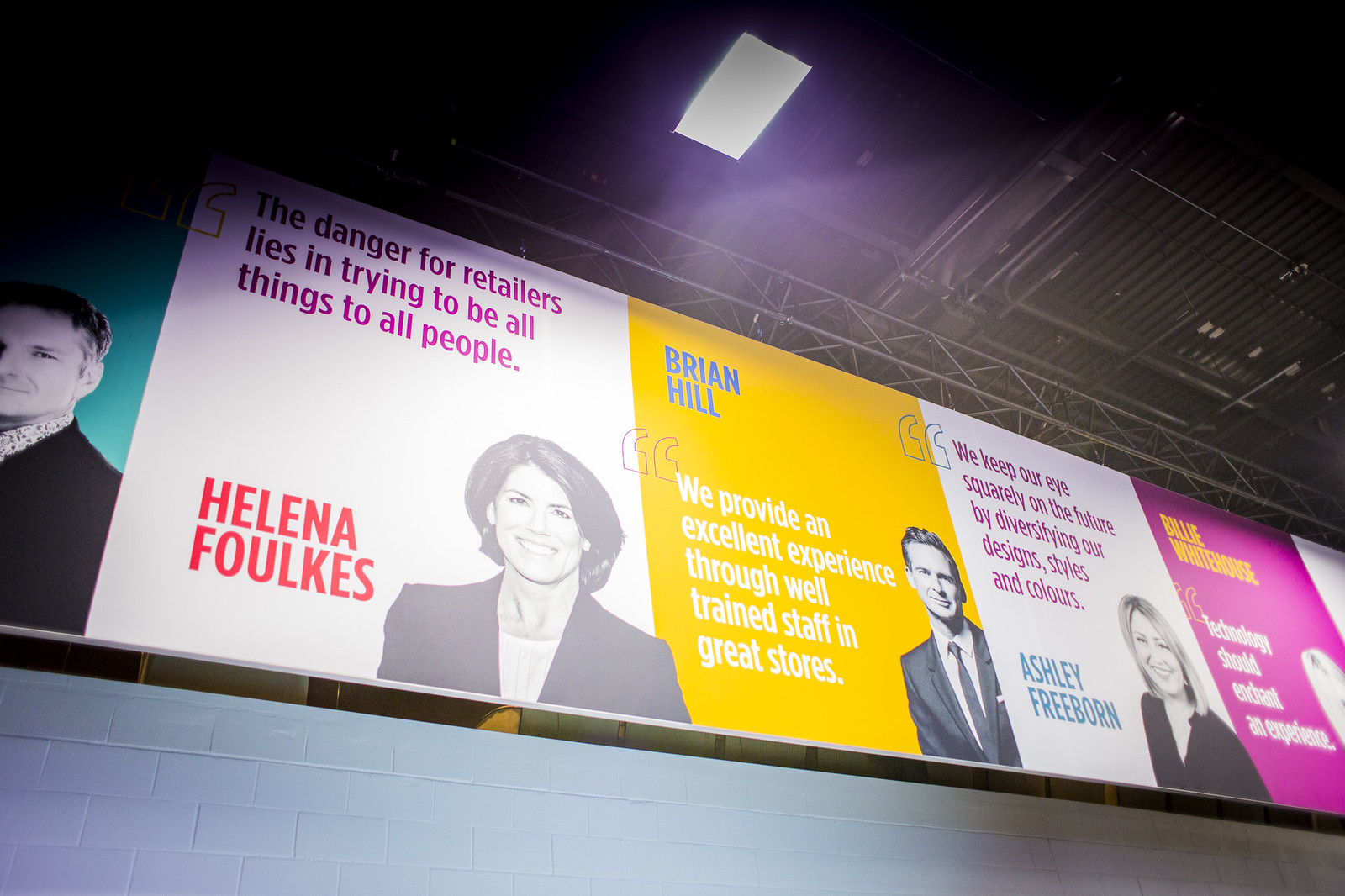This photograph, possibly taken inside a large warehouse-like building or train station, depicts a massive, top-down banner hanging against a black wall near the ceiling, which is illuminated by a skylight and spotlights. The ceiling features industrial elements such as metal pipes and walkways. The banner introduces several individuals, each in separate sections with their names, black-and-white photos, and quotes.

Starting from the left, partially cut off, is an image of a man whose details are not visible. Next to him is a section with a white background featuring Helena Foulkes. Her black-and-white photo is accompanied by her name and a quote that reads, "The danger for retailers lies in trying to be all things to all people." Adjacent to Helena's section, against a yellow background, is Brian Hill, a young man in his 20s. His quote, written in blue, says, "We provide an excellent experience through well-trained staff and great stores." Further to the right, another section with a light-haired woman named Ashley Freeborn showcases her quote: "We keep our eyes squarely on the future by diversifying our designs, styles, and colors." The final, partially visible section on the right appears to be bright purple, but its details are illegible. This detailed and illuminated banner highlights various figures and their insights, likely celebrating leadership or innovation in a professional setting.